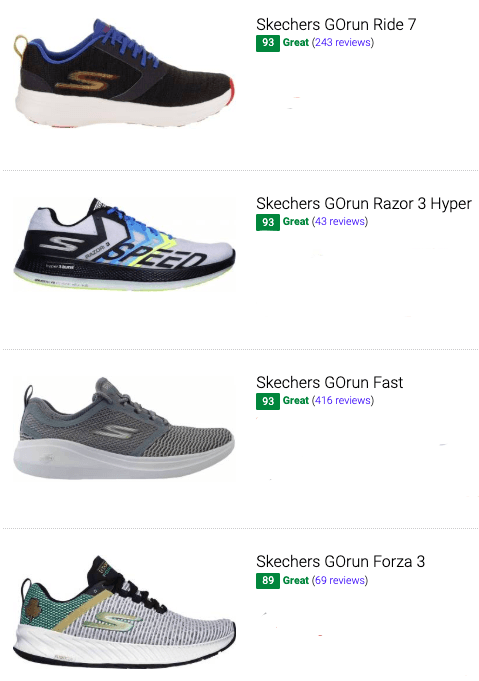**Detailed Caption:**

This screenshot showcases a comprehensive listing from a website that rates various Skechers running shoes. The header of the page prominently displays the top-rated Skechers shoes, each accompanied by a high-resolution, photorealistic image showing the side profile of the shoe.

1. **Skechers Go Run Ride 7:** This shoe tops the list with an impressive rating of 93, labeled as "Great" in green text. It has garnered 243 reviews, which are shown in purple.

2. **Skechers Go Run Razor 3 Hyper:** Also rated at 93 and marked as "Great" in green, this shoe has 43 reviews highlighted in purple.

3. **Skechers Go Run Fast:** Matching the top ratings, this shoe has a score of 93, noted as "Great" in green. It has received 416 reviews, which are indicated in purple.

4. **Skechers Go Run Forza 3:** Slightly lower in the ranking, this shoe has a rating of 89, still marked as "Great" in green, with 69 reviews shown in purple.

Each listing features clear, vivid images of the shoes, alongside their names, ratings, and the number of reviews, providing a detailed and helpful summary for potential buyers.